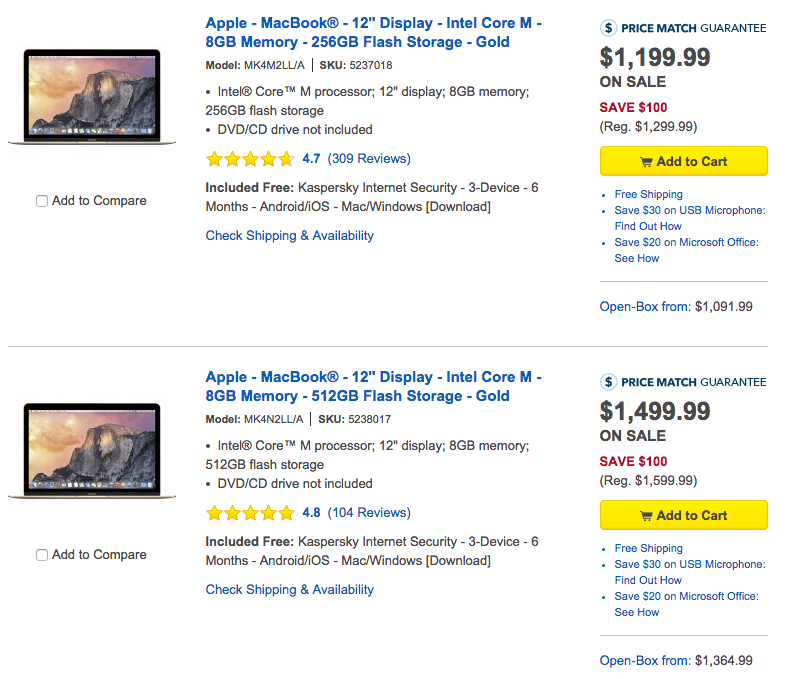Screenshot of a search result comparing two Apple MacBook laptops: 

**Top Result:**
- **Model:** Apple MacBook with 12-inch display
- **Processor:** Intel Core M
- **Memory:** 8 GB
- **Storage:** 256 GB flash storage
- **Color:** Gold
- **Price:** $1,199.99 (on sale, originally $1,299.99, save $100)
- **Reviews:** 4.7 stars from 309 reviews
- **Included Extras:** 
  - Kaspersky Internet Security (3 devices, 6 months; compatible with Android, iOS, Mac, and Windows)
- **Other Offers:** 
  - Save $30 on USB microphone (details on how to save available)
  - Save $20 on Microsoft Office (details on how to save available)
  - Open box option available from $1,091.99
- **Shipping:** Free shipping available
- **Purchase Options:** Add to cart

**Bottom Result:**
- **Model:** Apple MacBook with 12-inch display
- **Processor:** Intel Core M
- **Memory:** 8 GB
- **Storage:** 512 GB flash storage
- **Color:** Gold
- **Price:** $1,499.99
- **Reviews:** Identical offers as the top result
- **Open Box Option:** Available from $1,364.99
- **Shipping:** Free shipping available
- **Purchase Options:** Add to cart

Both models offer a detailed comparison primarily in terms of storage capacity and price, featuring bundled internet security software and additional promotional savings on accessories and software.